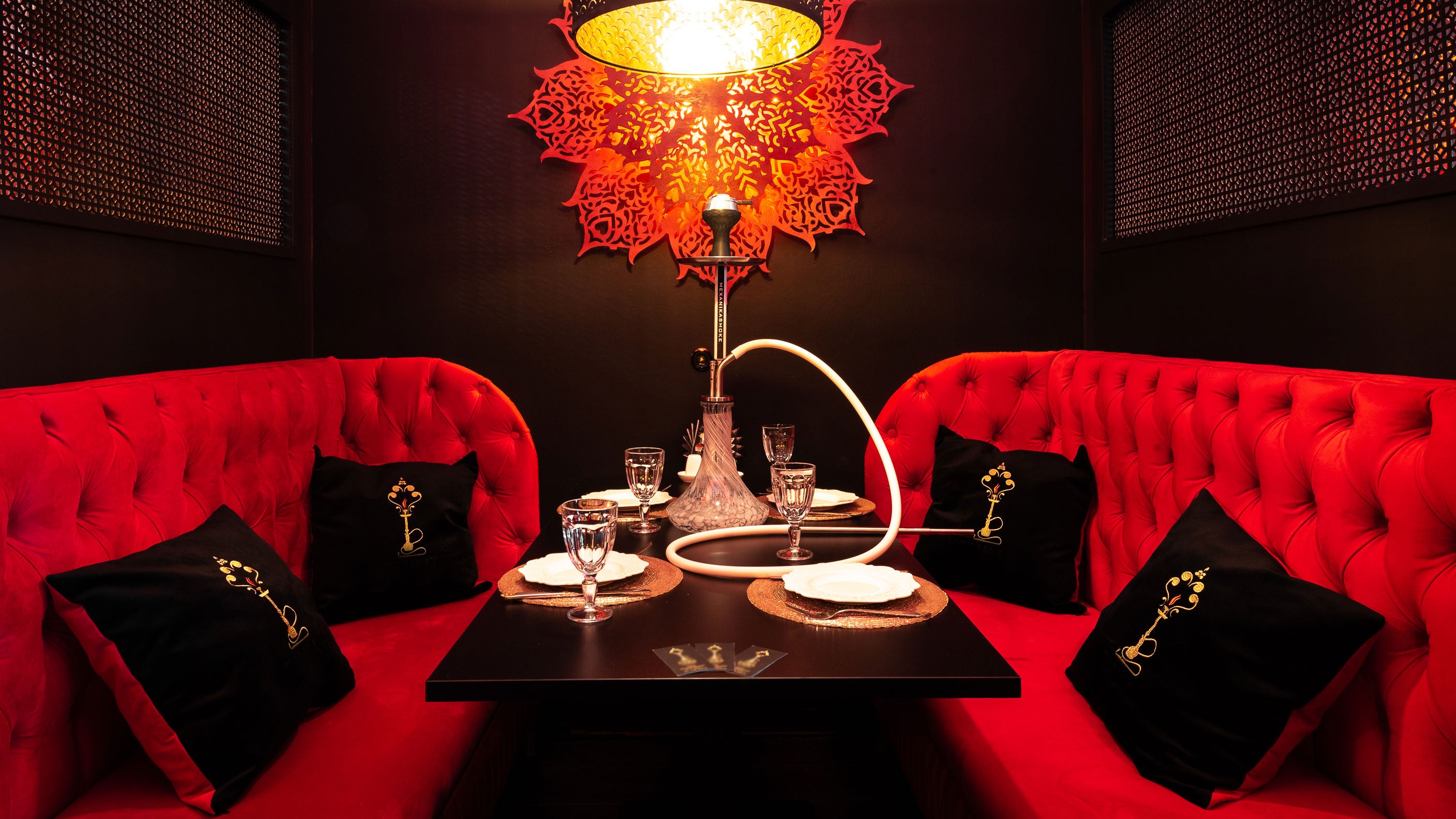This color photograph captures a cozy and inviting hookah lounge. At the center of the image is a dark brown, wooden table set with four plates and four clear wine glasses. A hookah with a pipe is prominently placed in the middle of the table. Surrounding the table on either side are two plush, deep red sofas, both of which feature dimpled backs and sides. Each sofa is adorned with two black throw pillows that have golden images of hookahs at the center. A warm, incandescent lamp hangs from the ceiling, providing gentle illumination to the setting. The room’s walls are entirely black, adding to the intimate and relaxing ambiance. A striking red decoration resembling a large lotus flower adorns the back wall, contributing to the aesthetic appeal of the space. Additionally, black grills are present on the top corners of the walls, extending across the width of the picture. This photograph beautifully captures the inviting atmosphere of this stylish and well-appointed hookah lounge.